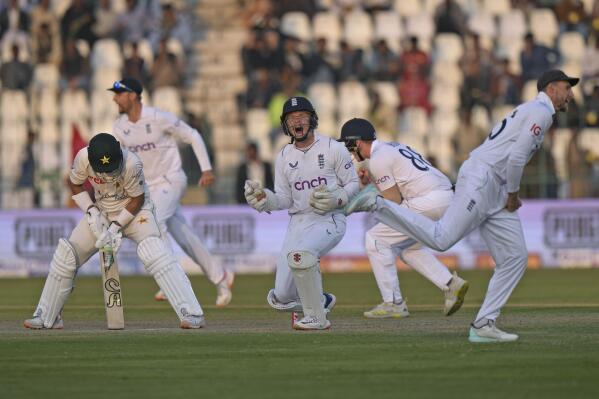The image captures a triumphant moment in a cricket game featuring five men celebrating an apparent victory on a green field. These athletes are clad in white uniforms, including long sleeve shirts, pants, and black helmets with face guards. One player, positioned on the far left, holds a cricket bat and is outfitted with knee guards, while the others either have gloves on or empty hands. The scene is vibrant with motion, as one player is seen running and another is down on one knee as they revel in their achievement. Behind them, a blurred crowd, dotted with individuals wearing red and blue, fills the stadium seats, though not to capacity. Less enthused than the players, these spectators create a subdued backdrop, alongside a blurry advertisement for PUBG. The collective excitement and the setting champion the moment of victory in this dynamic cricket scene.